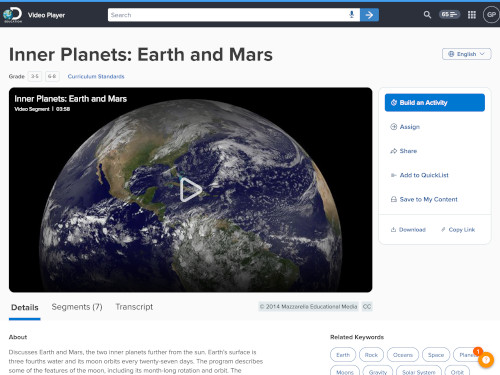The webpage resembles the Discovery Channel's layout, featuring the Discovery icon prominently in the upper left-hand corner. The "D" in the logo is backed by a rounded image of Earth, situated within a top navigation bar. To the right of the "Discovery" logo, there is a label reading "Video Player," followed by a search bar with a magnifying glass icon for search functionality. The profile of the logged-in user, indicated by the initials "GP," is displayed next to these elements.

Below the navigation bar, the title of the page reads "Interplanets: Earth and Mars." Beneath this title, there is a video section with a thumbnail image depicting Earth, and a play button centered within the image, all labeled as "Interplanets: Earth and Mars."

Underneath the video, users can access different sections titled "Details," "Segments," and "Transcripts." Additionally, a vertical menu is located on the right-hand side of the webpage.